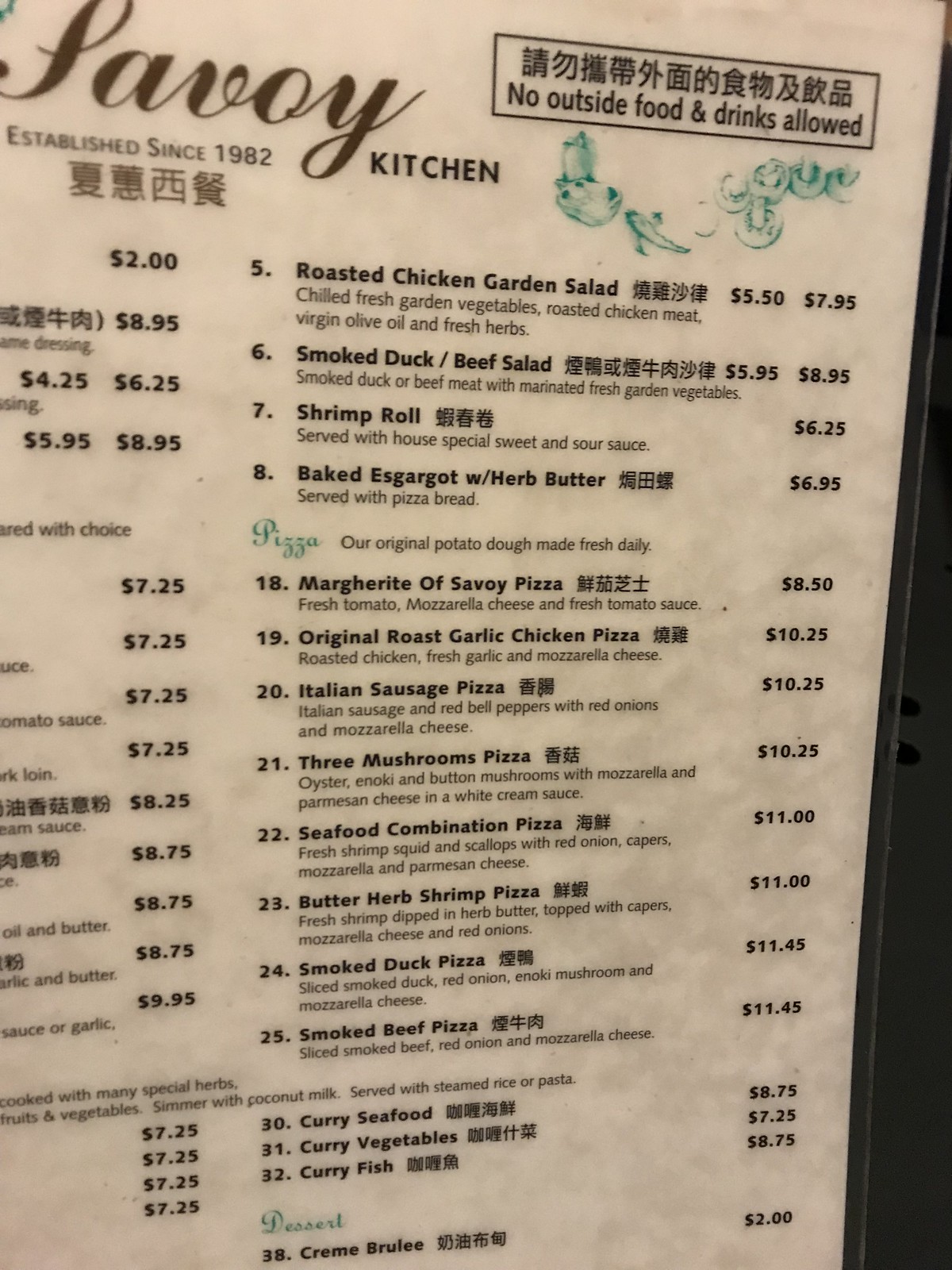The image features a restaurant menu with a sophisticated design. The background is a subtle off-white, and the text is presented in sleek black, punctuated with both English and Asian characters. The top of the menu showcases elegant green illustrations of vegetables, peppers, and mushrooms, providing an artistic touch. Centered at the top, the name of the restaurant, "Savoy," is written in refined cursive script, followed by "KITCHEN" in bold uppercase letters. Directly beneath this, "Established since 1982" appears, accompanied by more Asian characters.

The pricing information is listed along the left side of the menu, although the specific food items associated with these prices are not visible in the image. The displayed prices range from $2 to $8.95.

Dominating the right side of the menu are detailed food items and their corresponding prices:

- Roasted Chicken Garden Salad: $5.50 and $7.95
- Smoked Duck Beef Salad: $5.95 or $8.95
- Shrimp Roll: $6.25
- Baked Escargot with Herb Butter: $6.95

The menu highlights its pizza offerings in elegant green cursive, stating "Pizza." The accompanying description in black reads, "Our original potato dough made fresh daily." The selection includes:

- Margarita of Savoy Pizza: $8.50
- Original Roast Garlic Chicken Pizza: $10.25
- Italian Sausage Pizza: $10.25
- Three Mushrooms Pizza: $10.25
- Seafood Combination Pizza: $11.00
- Butter Herb Shrimp Pizza: $11.00
- Smoked Duck Pizza: $11.45
- Smoked Beef Pizza: $11.45

The curry section features:

- Curry Seafood: $8.75
- Curry Vegetables: $7.25
- Curry Fish: $8.75

The dessert section is introduced in green script with the word "Dessert," followed by the item's description in black:

- Crêpe Brûlée: $2.00